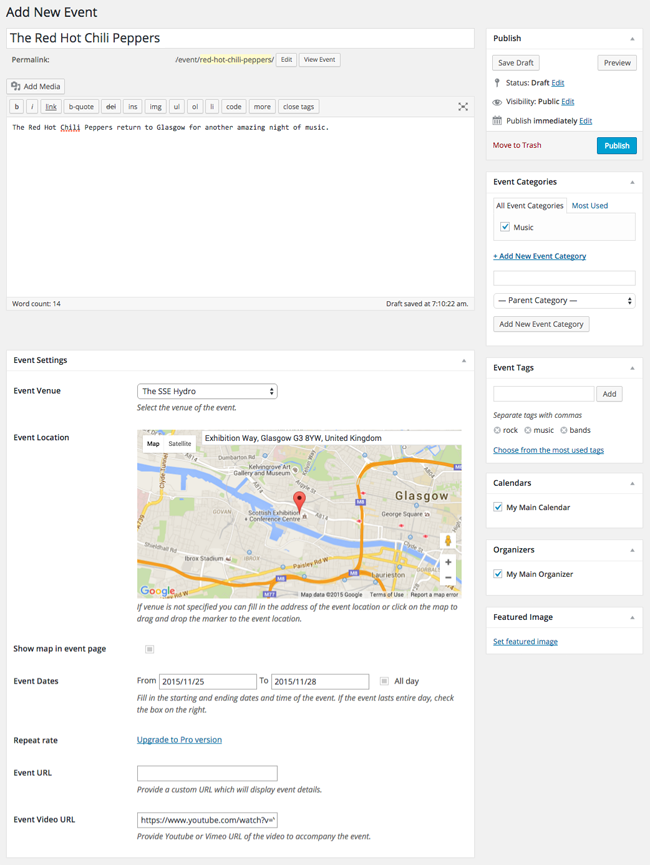Screenshot of a computer webpage for adding a new event. At the top, there is black text saying "Add New Event" inside a white rectangle. Beneath that, in black text, it reads "The Red Hot Chili Peppers". Below this text is a large white square containing some text, with the word "Chili" underlined in red in very small black text. 

Below the white square, there is an image of a map displaying the event location in the United Kingdom, indicated by very small letters that read "event location". On the right side of the page, there is an option to "Publish", and beneath that, a square button with text inside saying "Send a Draft". Slightly below this, in small red text, it reads "Move to Task". To the right of this, inside a blue rectangle, it says "Publish".

Further down within the content area of the white square, there are multiple sections consecutively labeled as "Event Categories", "Event Tags", "Calendars", "Organizers", and "Featured Image".